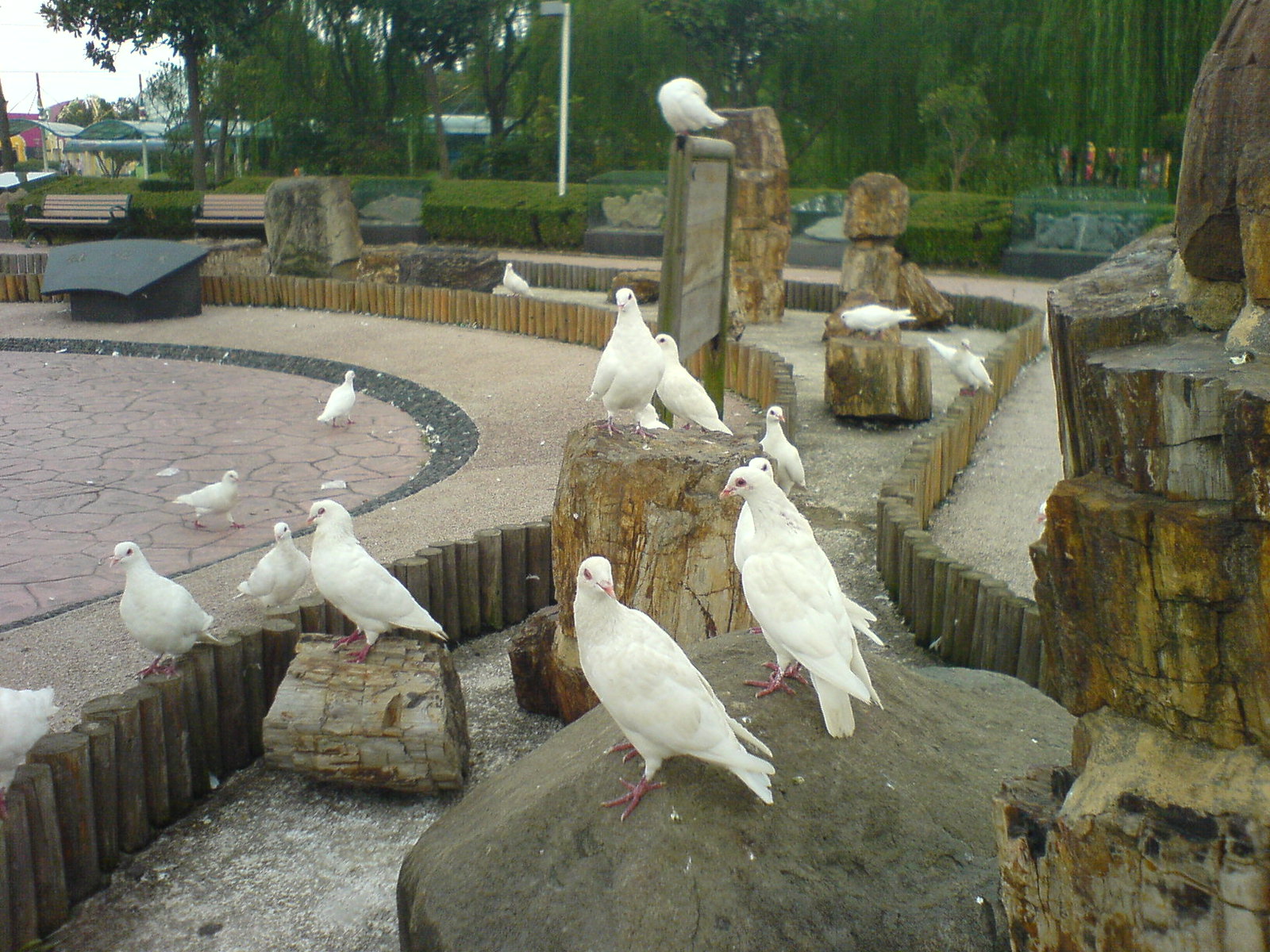In the foreground of this daytime image, a myriad of white doves with pink beaks and webbed feet congregate on the ground and perches. These perches are half-cut logs forming a low, brown wooden fence that outlines a park feature. The scene is filled with various structures, including large tree trunks, bricks, and small wooden and metal park benches. Scattered throughout, the white doves create a picturesque focal point alongside the rustic wooden sculptures and pathways.

Beyond this, a lush green expanse stretches into the distance, marked by several bushy trees, including a weeping willow suggesting the presence of water, possibly a pond or stream. A modest sign stands erected at the fence, host to another dove, while a series of oval-roofed structures and green awnings appear in the background, hinting at sheltered spots or picnic areas. Brown brick paths trimmed in black weave through the park, dotted with benches and providing areas for walking or possibly driving. The image captures a serene park crowded with 20 to 30 birds, bringing a lively charm to the natural and constructed elements of the scene.